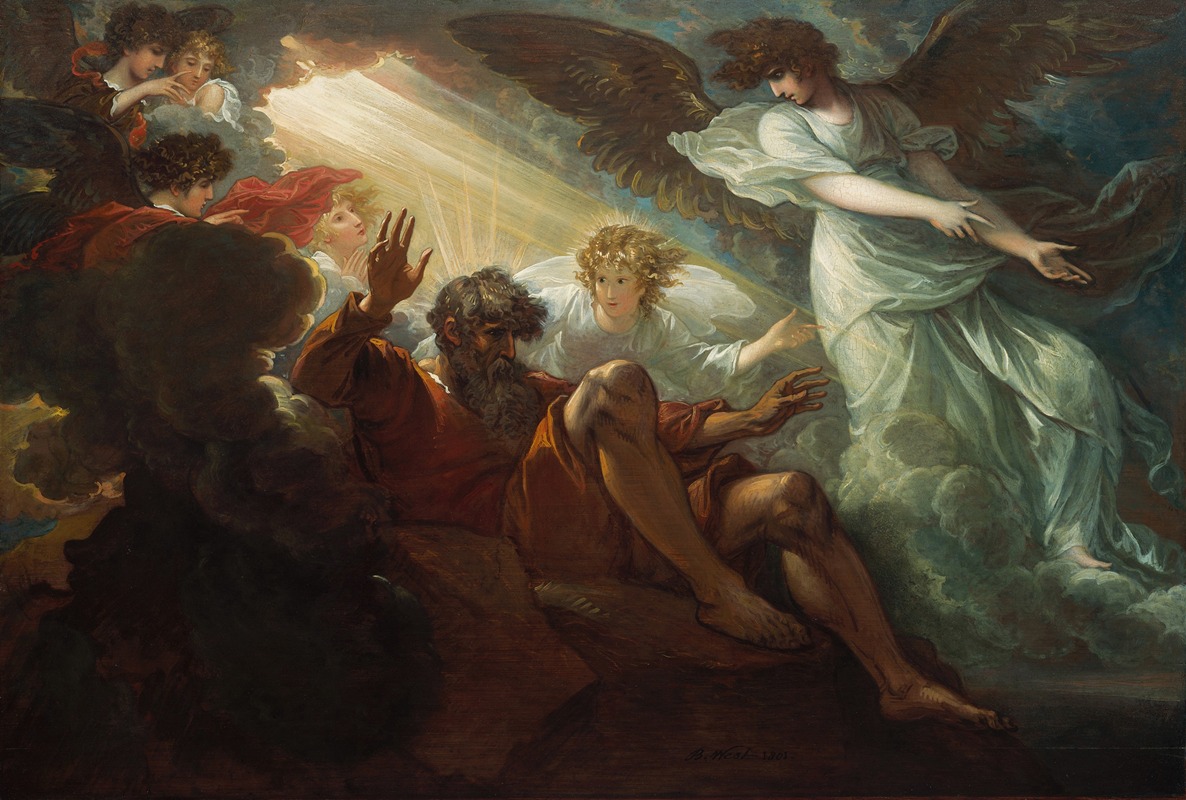The image vividly depicts a Renaissance painting, likely a ceiling mural, featuring a central figure interpreted as God. He is portrayed with long, bushy gray hair, a matching beard, and a mustache, clad in an orange-brown robe that drapes over his reclining form. Surrounding him are numerous angels, each adorned in flowing white gowns. The angels exhibit diverse wing types: some have pure white wings, while others possess larger, bird-like ones. Their hair varies from brown to blonde, and their skin is notably pale. Adding to the celestial scene, the sky above opens up to reveal sunlight piercing through clouds, creating an ethereal backdrop. The detailed arrangements and color palette—ranging from white, blue, and sky blue to hues of yellow, brown, and orange—accentuate the divine and historical essence of the painting.